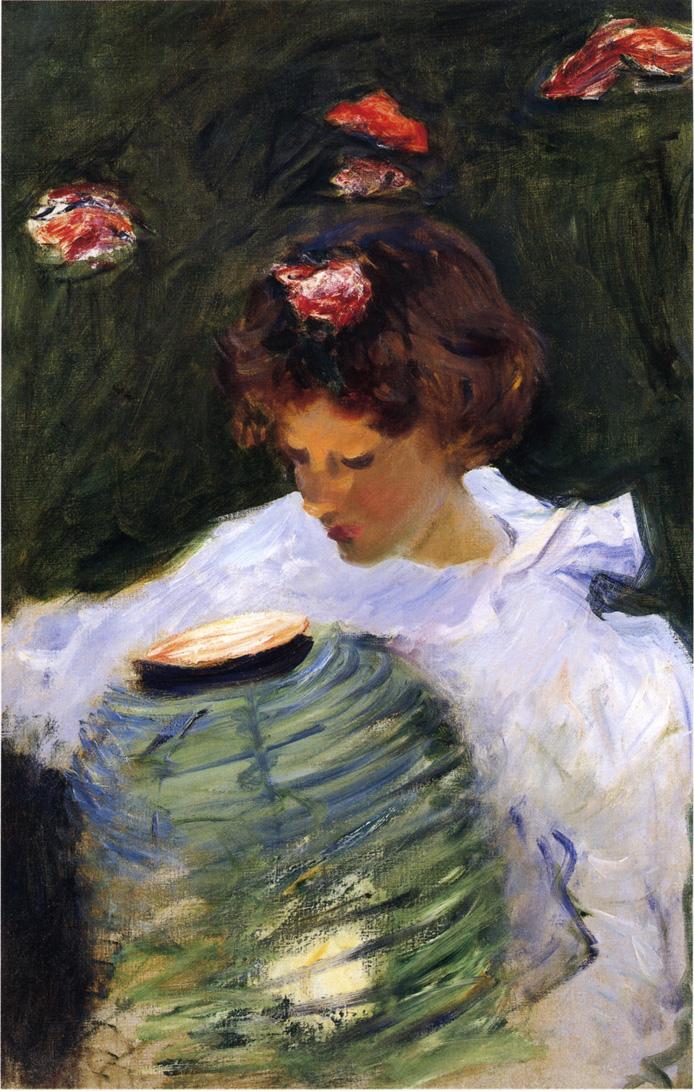The painting depicts a young woman with a tan complexion and short, pixie-like brown hair adorned with an abstract red and white flower. She is gazing downwards into a light green, swirling lantern that is illuminating her face. Clad in a simple white blouse, she stands against a background of muddled greens and browns, resembling an abstract tree or bush. The scene is accented by floating brush strokes of reds, yellows, and whites, which resemble leaves or ember-like elements adding a dynamic, almost ethereal quality to the composition. The overall atmosphere is dreamlike and richly layered with texture and color, bringing depth to the central figure and her enigmatic lantern.